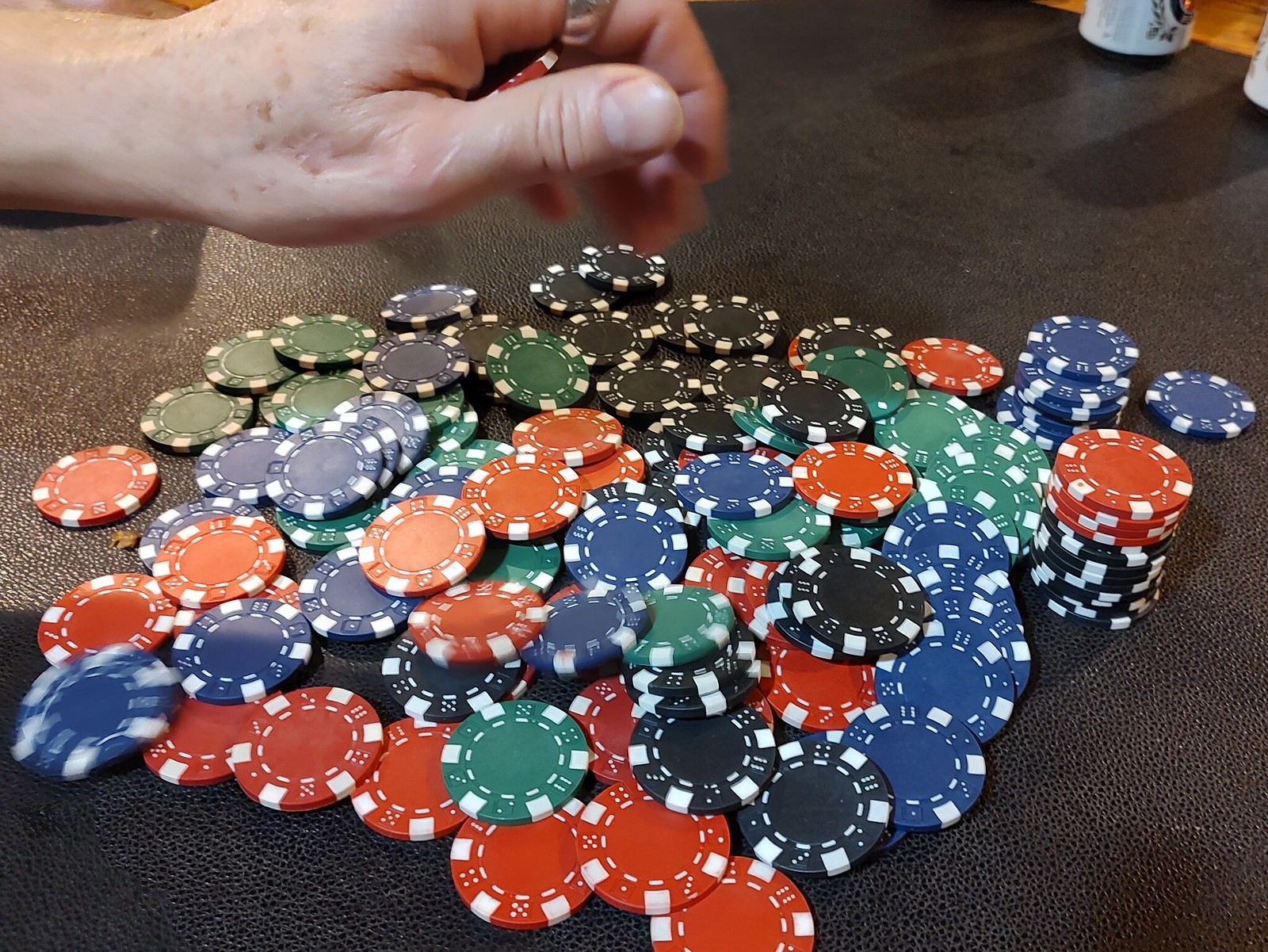A detailed color photograph captures a textured tabletop reminiscent of pebbled leather. Dominating the scene is an array of poker chips of various colors—red, green, black, blue, and white—effortlessly scattered across the surface. A pile of black and white poker chips sits on the right, crowned by a neat stack of four white chips. Just behind it stands another stack of blue and white chips, with a solitary blue and white chip lying nearby. Amidst this chaotic spread, an older hand, adorned with age spots and wearing a ring around the index finger, hovers near the top left corner. This hand clasps a red poker chip, seemingly in the act of placing it onto the crowded tabletop. In the upper right corner, two beer cans—one distinctly white with a laurel wreath design—peek into the frame, casting long, soft shadows across the scene, hinting at a relaxed, yet competitive atmosphere.